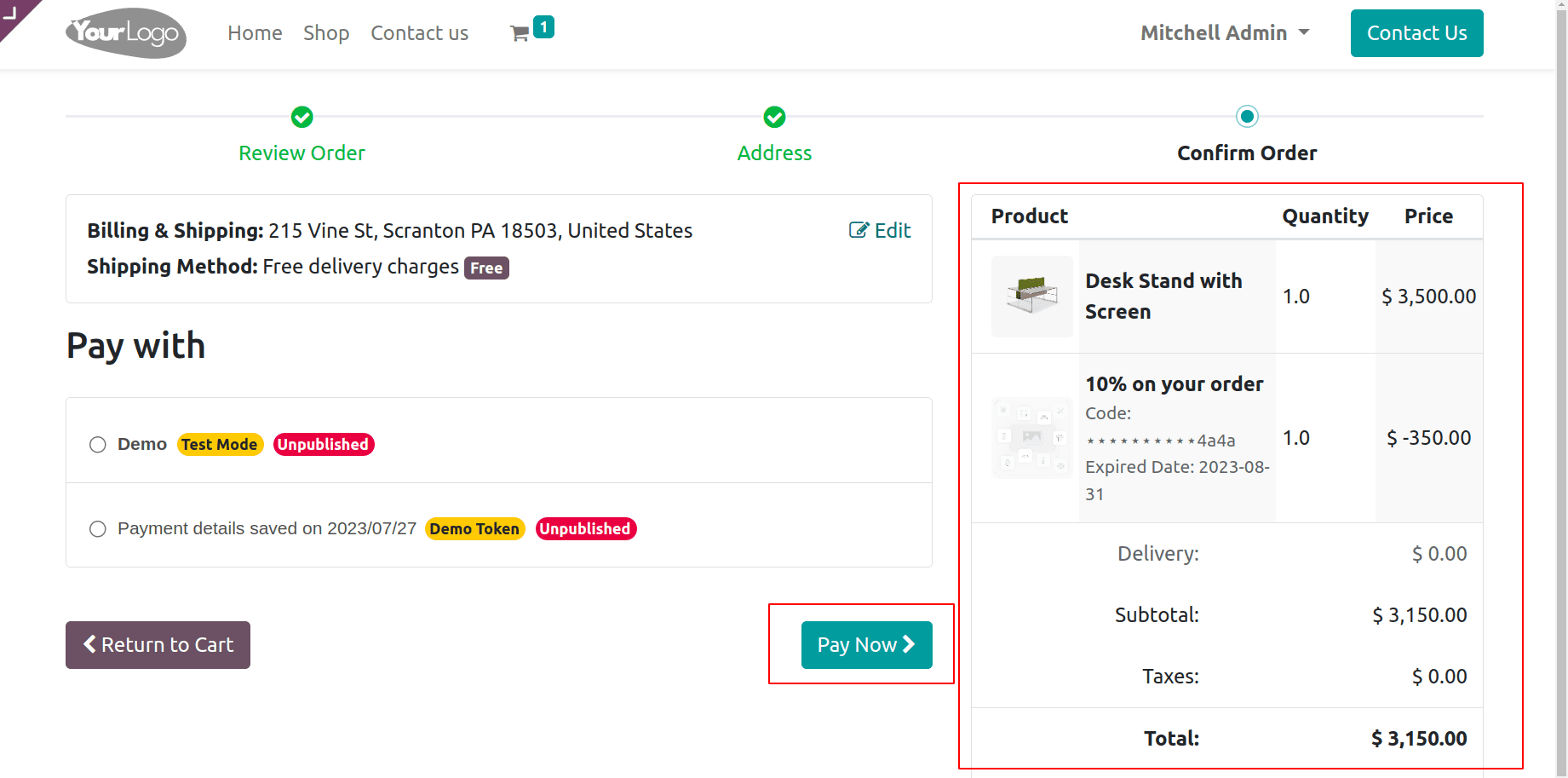**Caption**

This is an image depicting an invoice from an online shopping website. At the top of the webpage, there are standard navigation options including "Your Logo," "Home," "Shop," "Contact Us," and an icon showing a shopping cart containing one item. The main portion of the page is dedicated to the details of the transaction and shipping information.

The invoice addresses the customer at "2015 Vine Street, Scranton, PA, 18503, United States." It indicates that the shipping method selected was "Free Delivery," with no additional shipping charges. Payment details show the mode as "Demo," with the note "Payment details saved [2023-07-27]." The customer also has the options "Return to Cart" and "Pay Now."

Off to the right, the detailed breakdown of the order includes:
- **Product:** Desk Stand with Screen
- **Quantity:** 1
- **Price:** $3,500

The customer utilized a 10% discount code "4A4A" which was expired on "2023-08-31," resulting in a discount of $350. The item benefited from free shipping, bringing the subtotal to $3,150 and the total after taxes to $3,150.

In summary, the image shows a detailed invoice for an order comprising a desk stand with a screen initially priced at $3,500. The customer received a 10% discount and free shipping, with a final total amounting to $3,150.